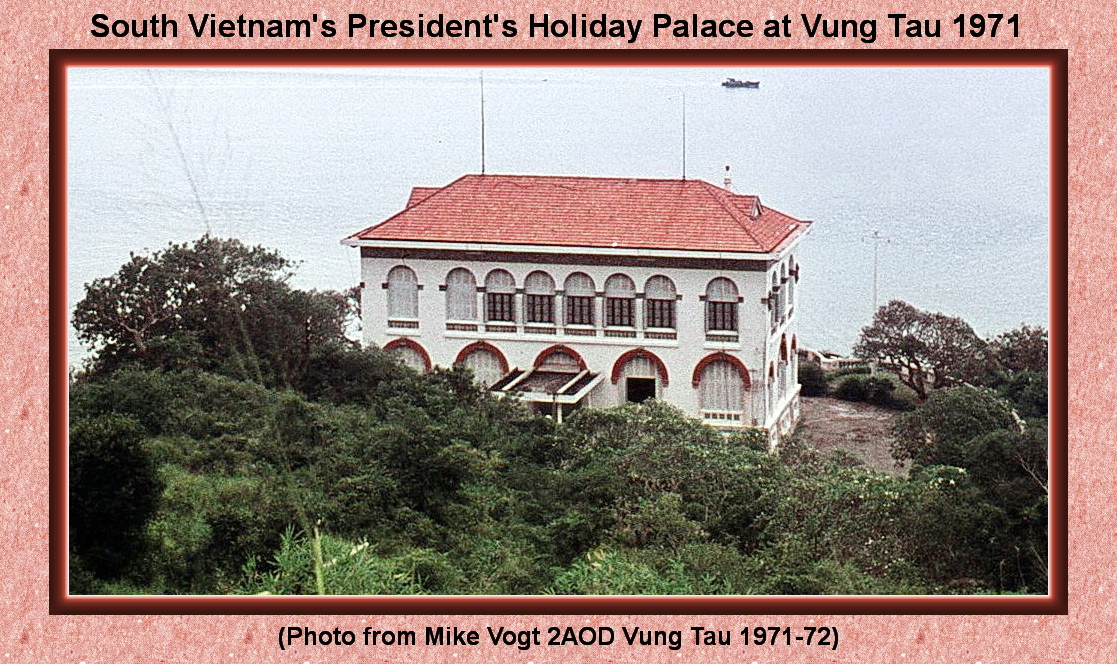The image showcases a historical photograph bordered by a peach-pink frame with black text. The text at the top reads "South Vietnam's President's Holiday Palace at Vung Tau, 1971," and at the bottom, it states, "Photo from Mike Vogt, 2nd AOD, Vung Tau, 1971-72." The picture is taken from an elevated perspective, possibly a hill or plateau, capturing a large, two-level, rectangular white building with distinctive red roofing and red accents around its windows and doors, reflecting the early French colonial architectural style prevalent in Vietnam. The building stands amid a lush, dense forest which leads to a clearing or driveway on the right side. Beyond the mansion, a serene body of water is visible, suggesting it may be the ocean or a significant waterway.